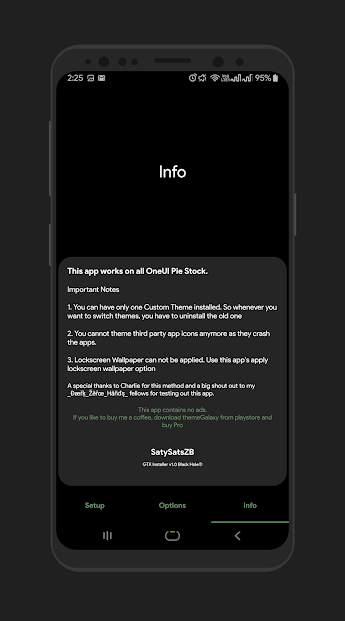The image features a simulated, computer-generated graphic of a smartphone on a gray background. The phone is oriented vertically and appears slightly smaller than a real-life smartphone, but still maintains a rectangular shape. The screen of the phone is primarily black with various standard icons at the top, indicating signal strength, battery percentage, and the current time.

Centered about a quarter way down from the top of the screen is the word "Info" displayed in white text. At around the halfway point of the screen, a gray square box occupies the space and extends almost to the bottom, leaving a slight gap above the navigation options.

Within this gray square, tiny white text provides detailed instructions and notes about an app. The text reads:

"This app works on all One UI Pie stock or PLE stock. Important notes: 
1. You can have only one custom theme installed at a time. To switch themes, you must uninstall the old one. 
2. You cannot theme third-party app icons anymore as it causes the apps to crash.
3. The lock screen wallpaper cannot be applied directly; use this app's 'Apply Lock Screen Wallpaper' option.
Special thanks to Charlie for this method, and a big shout out to my [unreadable name] fellows for testing out this app."

Beneath this text, in green, it states: "This app contains no ads. If you like it, buy me a coffee. Download Theme Galaxy from the Play Store and buy Pro." In white text below that, it reads "Sadie sat or SATY SATZB" [exact text unclear].

Finally, at the very bottom, navigation options are displayed horizontally with labels such as "Setup" (centered), along with additional options and info on the left.